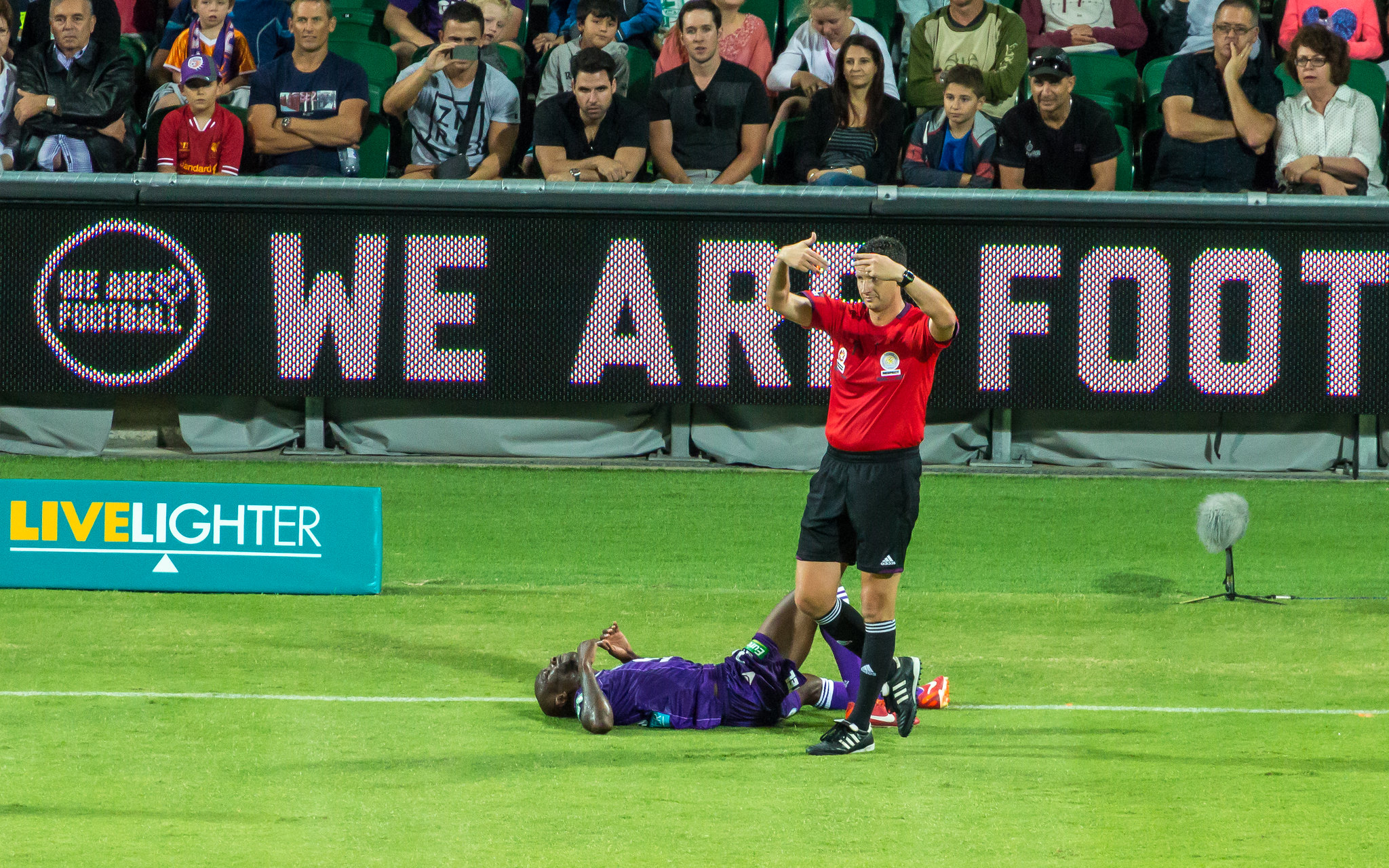The photograph captures an intense moment from an outdoor soccer match. At the forefront, an African-American male player lies on the green grass, appearing to be in pain. He has a bald head and is dressed in a purple uniform consisting of a purple shirt and shorts. Next to him stands a man in a red shirt and black shorts, along with black socks and Adidas cleats. The man in red, likely a player or referee, has his hands raised above his head as he observes the scene.

In the background, there's a stadium filled with multiple spectators watching the ongoing game. A prominent black banner is visible, partially reading "We Are Football," though only "We Are Foot" is fully visible due to the cropping of the image. Additionally, there is a turquoise-colored banner on the side of the field with the words "Live Lighter" printed on it; "Live" is in yellow, and "Lighter" is in white. This image effectively conveys the tension and atmosphere of the match, focusing on the players and the vibrant stadium environment.